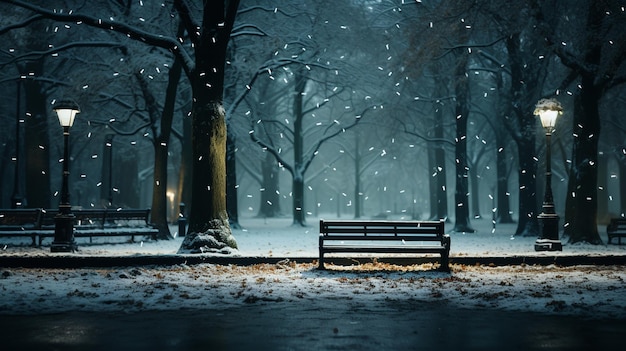This hyper-realistic digital painting depicts a serene nighttime winter scene in a park. Dominating the foreground is an empty bench slightly offset to the right, set against a curb that transitions to a street or parking lot. Scattered snow covers the ground, mingling with autumn leaves, while thicker snow adorns the park itself. The soft sky glows with falling snowflakes, enhancing the tranquil ambiance. Large, bare trees with thick, wide trunks stretch across the background, indicative of a heavily forested area. Two street lamps on either side of the image illuminate the walkway and add a warm contrast to the otherwise cold scene. Additional benches and lights can be spotted in the distance, adding depth to the composition. The overall effect, accentuated by the lighting and shadow play, emphasizes the central bench and the peaceful, snowy landscape surrounding it.